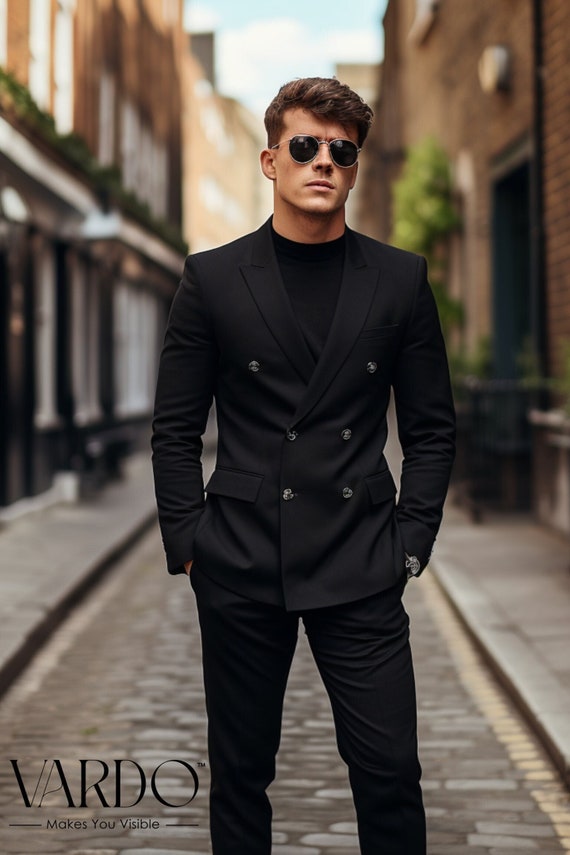In this captivating fashion photography ad, a stylish young man stands confidently on a narrow, European-looking cobblestone street, reminiscent of an elegant alleyway adorned with tall brick buildings and decorative awnings. The serene background, slightly blurred to enhance the focus on the model, features charming storefronts and colonial-style architecture with shrubbery adorning some walls. The model, a Caucasian male with short, meticulously styled brown hair and a chiseled jawline, exudes sophistication. He's clad in a sleek, all-black ensemble, consisting of a crew-neck t-shirt and a double-breasted suit jacket with shiny buttons, paired with matching black pants. Completing his suave look, he sports aviator sunglasses and a silver watch, with both hands casually tucked into his pants' pockets. The ad text in the foreground reads "Fardo TM" along with the tagline "Makes you visible," positioned thoughtfully on the left side. The overall setting and the model’s poised demeanor suggest this image is intended for a high-end fashion magazine or advertisement.